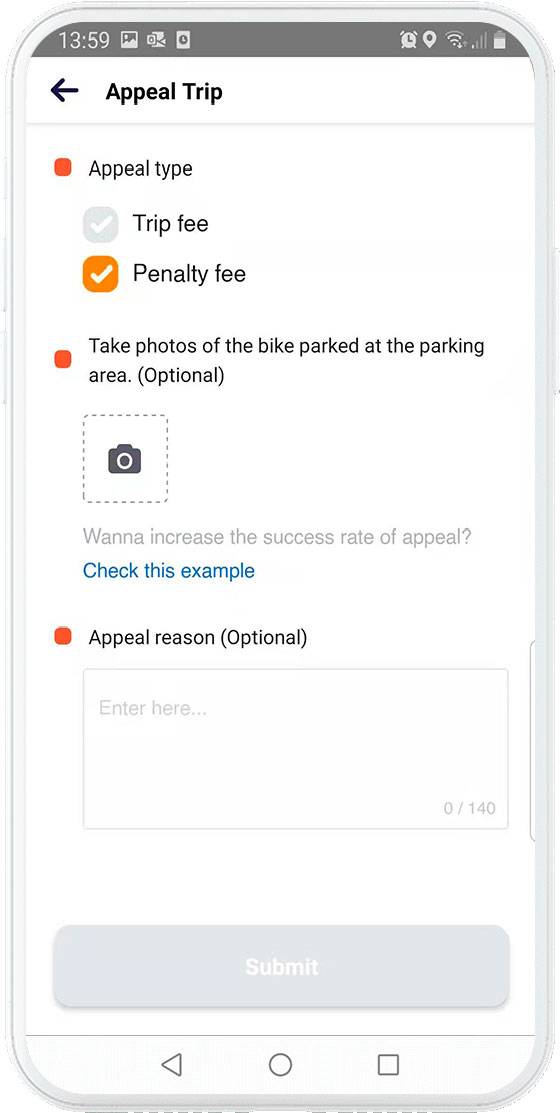This image is a screenshot of a smartphone's display at 1:59 PM, indicated by the digital clock reading "13:59" at the top. The status bar reveals several icons: an alarm notification, a location service icon, and various unseen emojis. The phone is connected to a Wi-Fi network with three bars, has only one bar of cellular service, and the battery is approximately 75% charged.

The main content appears to be a webpage, possibly related to some sort of service appeal process. At the top of the page, an arrow is seen overlaid on the words "Appeal Trip." Below this header, there's an interface for selecting an appeal type, with options for "Trip Fee" and "Penalty Fee." The "Trip Fee" option is grayed out, while the "Penalty Fee" is selectable, marked by an orange box with a white checkmark inside.

Further down, there is an instruction in a dark orange box stating, "Take Photos of the Bike Parked at the Parking Area," which is noted as optional. Adjacent to this instruction is a clickable camera emoji for uploading a photograph. Accompanying guidelines encourage users to increase the success rate of their appeal by checking examples.

At the bottom, another orange box labeled "Appeal Reason" allows for optional input, presenting a field where users can enter their explanation or comments.